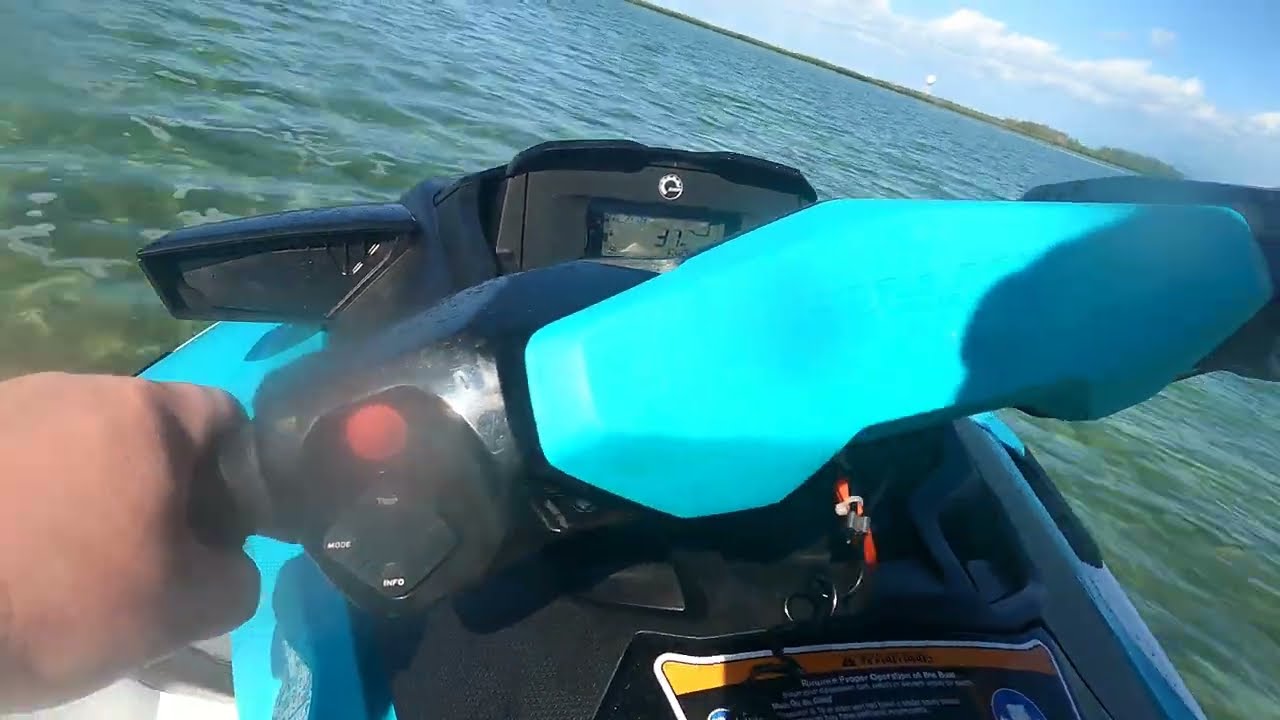The photograph captures a vibrant outdoor scene from the perspective of someone riding a jet ski on the ocean. The jet ski, primarily blue and black, prominently displays its left handlebar gripped by a slightly blurry hand of Caucasian descent. The handlebar, outfitted with a red ignition button and labeled buttons for "mode" and "info," sets the stage for the rider’s control. Just beneath the handlebar is an orange key nestled in the ignition. Above, a speedometer reads "37," indicating the speed. The entire viewpoint is slightly askew, suggesting a leftward turn, which tilts the horizon line diagonally from the top center to the right edge of the image. The ocean's water glimmers with a greenish hue, reflecting the clear blue sky above, dotted with a few clouds. Further in the background, the distant shoreline adds depth to the composition, encapsulating the essence of a thrilling ride under the open sky.